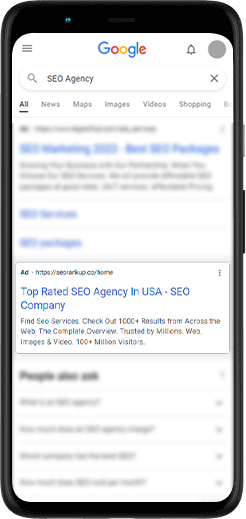A detailed screenshot depicts a Google search results page for "SEO agency." In the top-left corner, familiar icons include the Google logo and a hamburger menu symbol. To the right, there's a notification bell. Beneath this, the search bar contains the query "SEO agency" with an "X" on the right side to clear the input, and a magnifying glass icon on the left to initiate the search.

Below the search bar, there are various search category tabs: "All," "News," "Maps," "Images," "Videos," and "Shopping." The first section of results includes a website link with some additional information, followed by two adjacent links with minimal text. An advertisement appears immediately beneath this, promoting a top-rated SEO agency in the USA, featuring claims such as "SEO company bond," "SEO services," and highlighting over a thousand results from sites across the web.

Further down, there is a "People also ask" section with additional questions related to SEO. Another ad is prominently displayed, outlining offerings like complete SEO overviews, trusted by millions, with web images and videos catered to over 100 million visitors. This ad is encapsulated in a delineated rectangle, and in the top-right corner of this rectangle, three vertical dots indicate additional options.